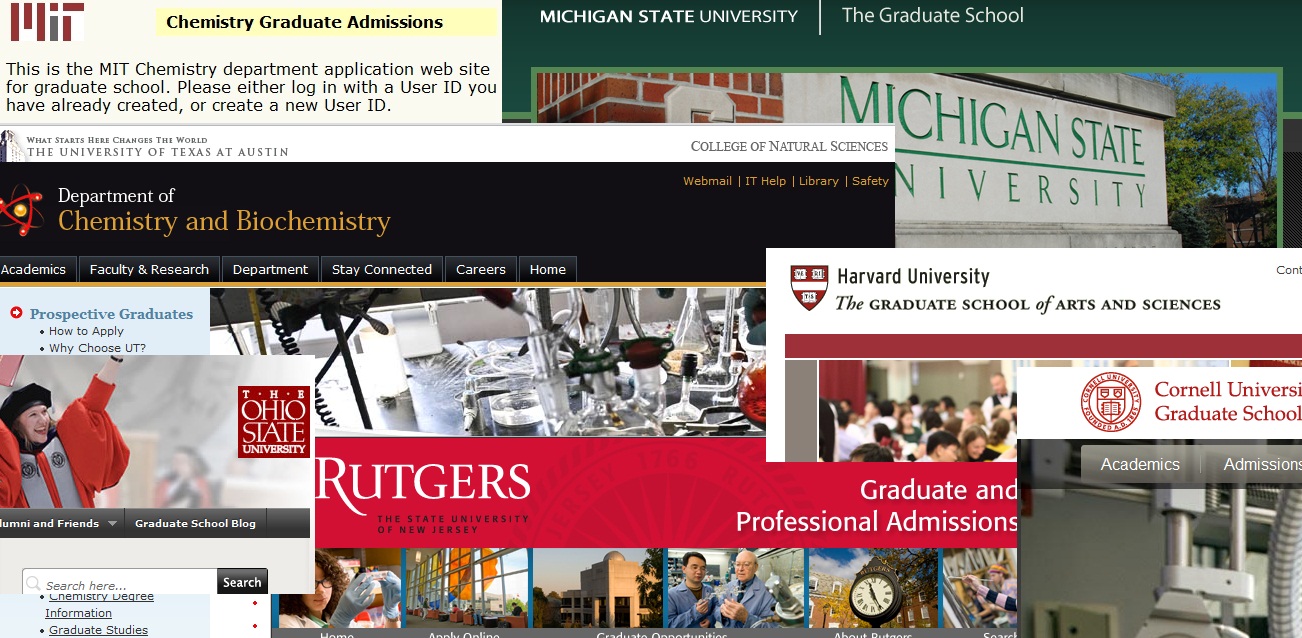This image is a screenshot of a web page featuring a collage of graduate school admissions information from various universities. At the very top, there are lines that form an abstract representation of the letters "MIT," followed by the text "Chemistry Graduate Admissions." This confirms that the web page is related to the Massachusetts Institute of Technology (MIT) Chemistry Department’s application for graduate school, prompting users to log in or create a new user ID.

In the middle and right side of the screenshot, there is text and an image related to Michigan State University. The visual depicts a brick building and a sign that reads "Michigan State University," with trees visible on the right side.

Overlapping with this, additional university information is presented, including:

- The University of Texas at Austin, College of Natural Sciences, Department of Chemistry and Biochemistry, with the tagline "What starts here changes the world."
- The Ohio State University, featuring a graduate school blog.
- Rutgers, The State University of New Jersey, highlighting graduate and professional admissions.
- Harvard University, showcasing its Graduate School of Arts and Sciences.
- Cornell University Graduate School.

Overall, the web page shows a collage of various prestigious university graduate programs, emphasizing their respective chemistry and biochemistry departments.